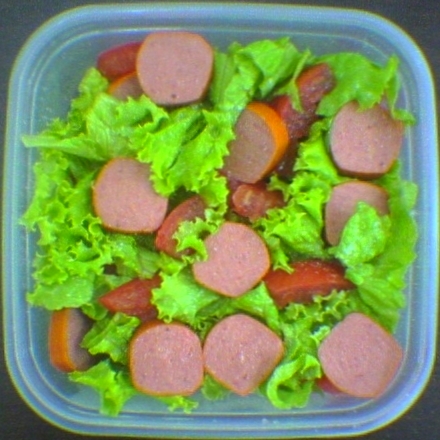The image shows a top-down view of a clear blue, square Tupperware container with rounded corners, filled with a vibrant, freshly-washed salad. The salad consists of bright green loose-leaf lettuce, which remains whole rather than chopped. Scattered throughout the lettuce are slices of sausage or hot dog, light brownish-pink in color, with an orange ring indicative of the sausage casing. There are approximately eight or nine visible circular slices of this sausage. Additionally, among the greens are several bright red, chopped tomato chunks, adding a splash of color and contrast to the mix. The tomatoes are visibly juicy, with tiny seeds discernible in their centers. The simple yet colorful and fresh composition fills the entire container, making for an appetizing and wholesome presentation.